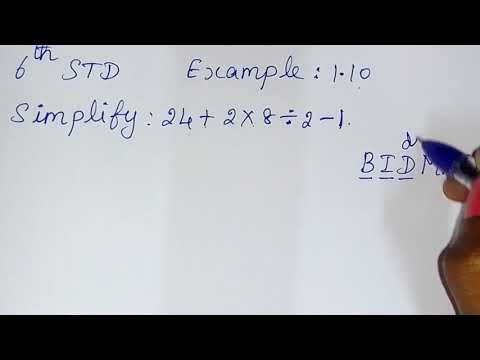The image depicts a close-up shot of a hand holding a blue pen, poised to write on a sheet of white paper. The hand, with visible fingers on the right side, one of which has pink nail polish, is casting a slight gray shadow over the paper. The pen is in the process of writing the lowercase letter "d." At the top left of the page, it reads "6th STD example: 1 through 10" in a blend of cursive and lowercase print. Below that, there is a mathematical expression written in blue ink: "Simplify: 24 + 2 × 8 ÷ 2 - 1." The letters "BIDM" appear underneath, with most of the letters underlined except for the last character, which is partially obscured by the pen. The image captures the moment just as the pen touches the paper to complete the writing.